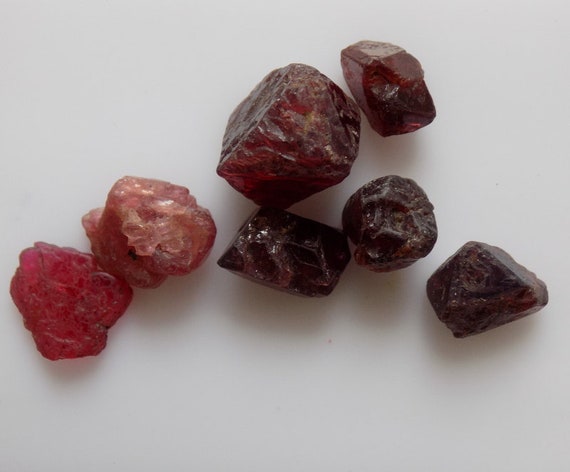The photograph features seven unpolished gemstones arrayed on a white background, possibly a table or piece of paper. The stones are mid-sized, easily fitting into the hand, and exhibit a range of hues from bright red to deep purplish-red. On the left, two stones display a vivid red and pinkish hue, with one appearing particularly flat and somewhat squashed. To the right, five stones transition into darker shades of maroon, brown, and deep wine-red, with a subtle translucent quality. Their surfaces vary in texture, with the left stones being more jagged and the right ones smoother and rounder. These raw, uncut stones, potentially rubies, spinels, or garnets, bear the natural beauty typical of specimens destined for a museum exhibit.